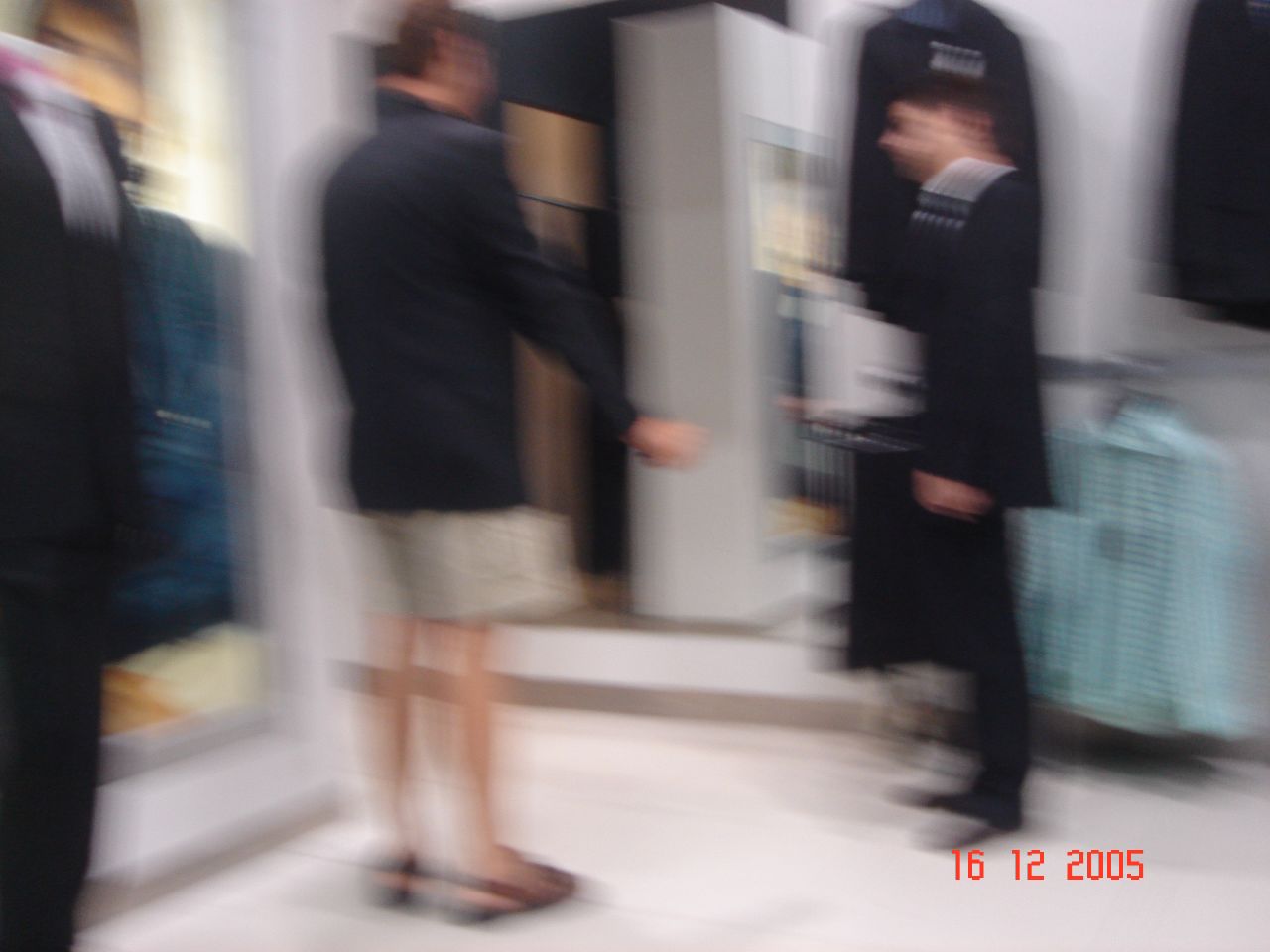In an extremely blurry photograph, timestamped in red "16-12-2005" at the bottom right, the scene depicts the interior of what appears to be a store, suggested by clothing racks in the background. The setting features a white floor and predominantly white or off-white walls, creating a soft-lit ambiance. In the foreground, we observe two individuals conversing. The person on the left is a man dressed in tan cargo shorts, brown sandals, and a dark long-sleeve shirt, with brown hair. The individual on the right donning a full black suit appears to also have a white shirt and possibly a black hat. Their faces and movements are obscured by significant motion blur, adding a sense of mystery to the scene.